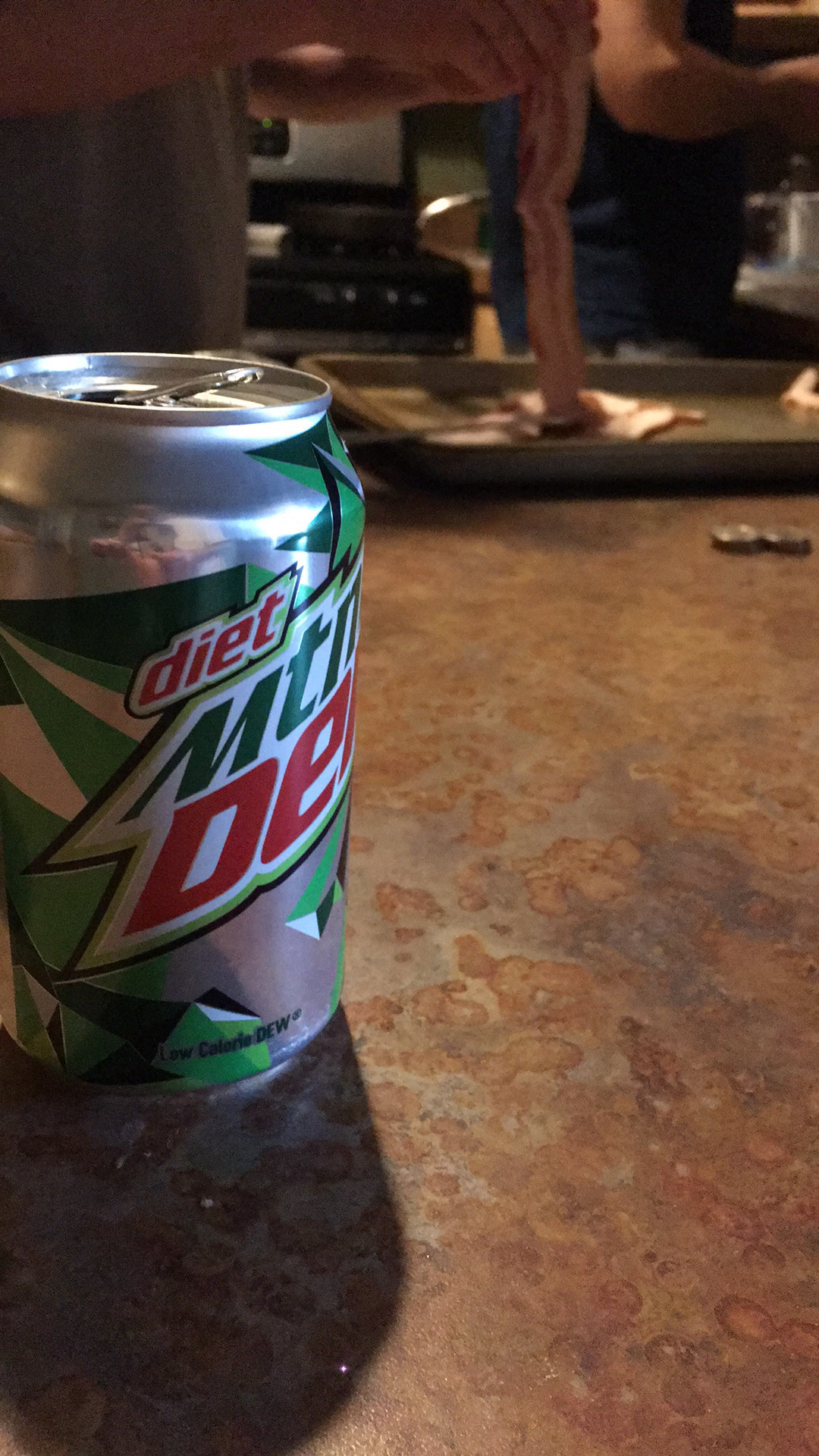This photograph features a close-up of an open Diet Mountain Dew can, prominently displaying the words "Diet Mountain Dew" in a mix of red, white, and green lettering. The can, mostly silver with patches of green, sits on a distressed brown surface, which appears to be a kitchen counter. In the background, a person wearing a black shirt is partially visible, identified by their elbow and hand as they manipulate strips of bacon, some of which are already placed in a pan. Additional kitchen elements are discernible, including a chair and the front of a range hood, hinting at a bustling cooking scene.